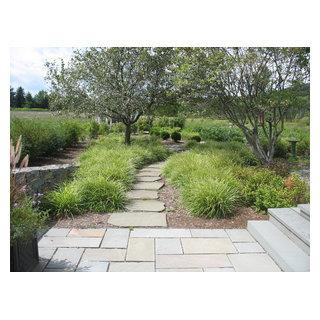The photograph captures a tranquil park or natural habitat on a partly cloudy day, with a light blue sky and white clouds peeking through tall green trees in the background. The foreground to the right is dominated by gray steps that lead down toward gray stone pavers. Larger stone steps run from the foreground to the background, flanked by gravel, dirt, and small bushes. To the left, there's a mix of shrubbery and a distinctive orangish-pinkish plant with the stone wall appearing further left. This serene scene features trees with lush green leaves and circular grassy bushes, all contributing to a calming and natural ambiance. The overall setting suggests a meticulously maintained landscape designed to evoke peace and tranquility.